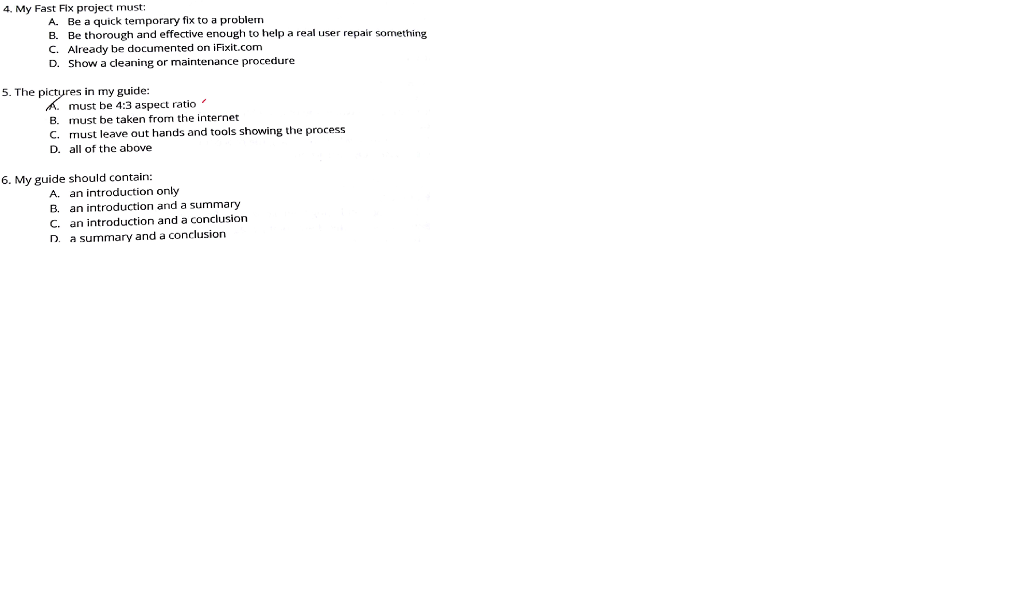This image appears to be a partial, cropped photograph possibly taken from a document. The background is solid white, emphasizing the content of the document. The image displays a list structure, focusing on three main sections labeled four, five, and six. The document seems slightly angled, with the text skewing upwards from left to right.

Section four, titled "My fast-paced project must:", lists requirements from A to D. Item A states "be a quick, temporary fix to a problem," while item D mentions "shut down a cleaning or maintenance procedure."

Section five, labeled "The pictures in my guide must:", suggests formatting instructions. Item A, although partially obscured, appears to specify a "three aspect ratio." This section seems to include items B and C, but they are cut off in the image.

The final section, number six, is titled "My guide should contain:". It starts with "an introduction only" and ends with "a summary and a conclusion."

Overall, the document seems to outline project and guide requirements, providing detailed and specific instructions under each numbered section.